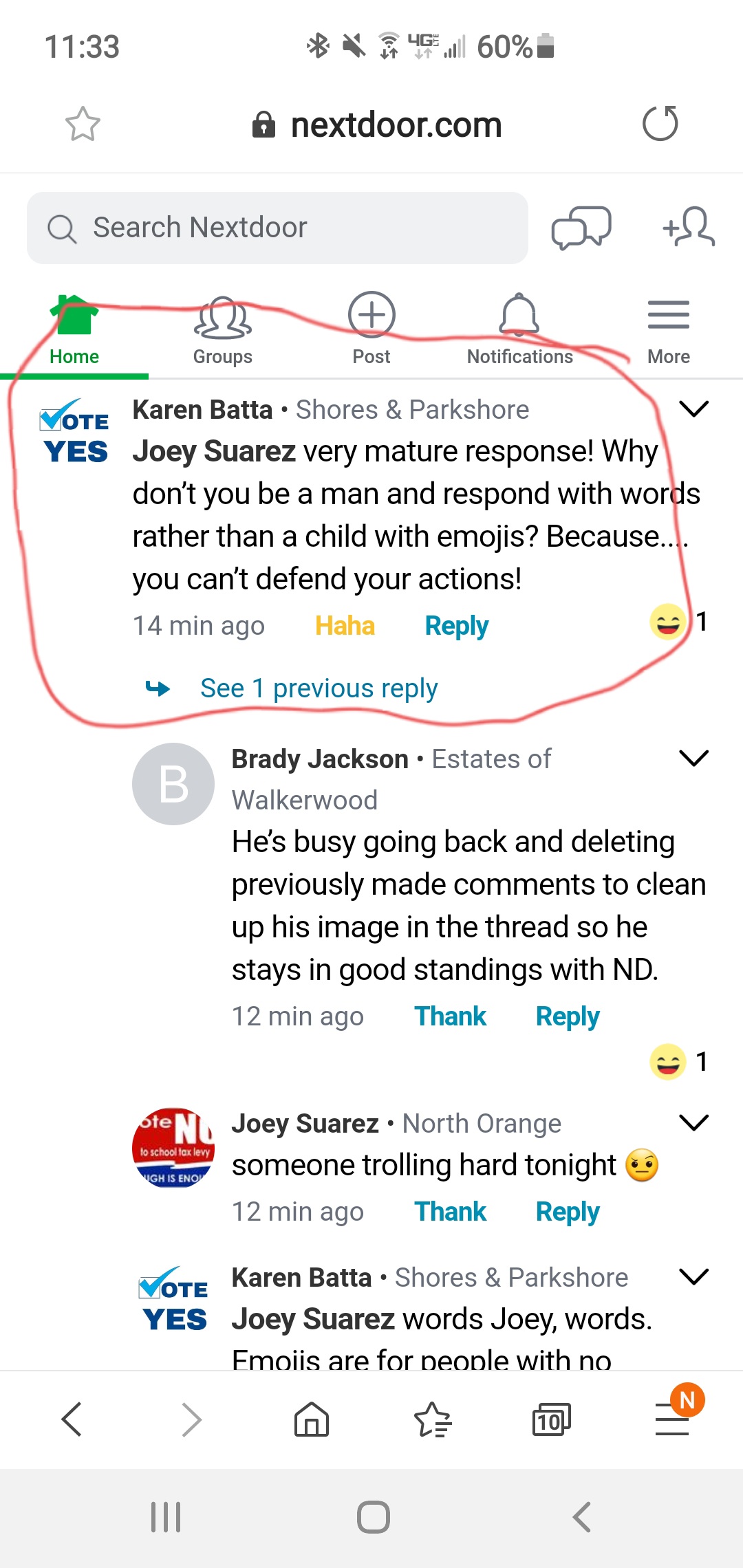Image Description: The screenshot appears to be from the mobile app of nextdoor.com. At the top of the interface, the word "nextdoor.com" is prominently displayed, indicating the platform. A search bar accompanies the header, allowing users to "Search Nextdoor." To the right of the search bar, there are two icons: one resembling a message bubble, and another depicting a person with a plus sign, suggesting user interactions like messages and friend requests.

Below the header, a navigation bar lists tabs such as Home, Groups, Post, and Notifications. Currently, the Home tab is selected, highlighted in green, while the others remain plain white. 

The main section of the screen displays a series of user interactions. Karen Bada, located at Shores and Park Shores, initiates a thread. In response, Joey Suarez comments critically, stating, "Very mature response. Why don’t you be a man and respond with words rather than a child with emojis because you can’t defend your actions." Below his comment, there are options to vote "yes," laugh ("ha ha"), or reply, with one previous reply partially visible but not fully shown.

Brady Jackson adds to the thread, noting that "he's busy going back and deleting previously made comments to clean up his image in the thread so he stays in good standings with N.D." Joey Suarez replies again with "Someone trolling hard tonight," accompanied by a neutral face emoji. Karen Bada chimes in once more, saying, "Joey, words; emojis are for people with no," but her comment is cut off.

At the bottom of the screen, typical mobile navigation icons are present, including a home button, a star icon, a multitab icon indicating several open pages, and a back arrow.

This detailed description encapsulates the essence of the interaction and the structure of the nextdoor.com mobile interface as displayed in the screenshot.